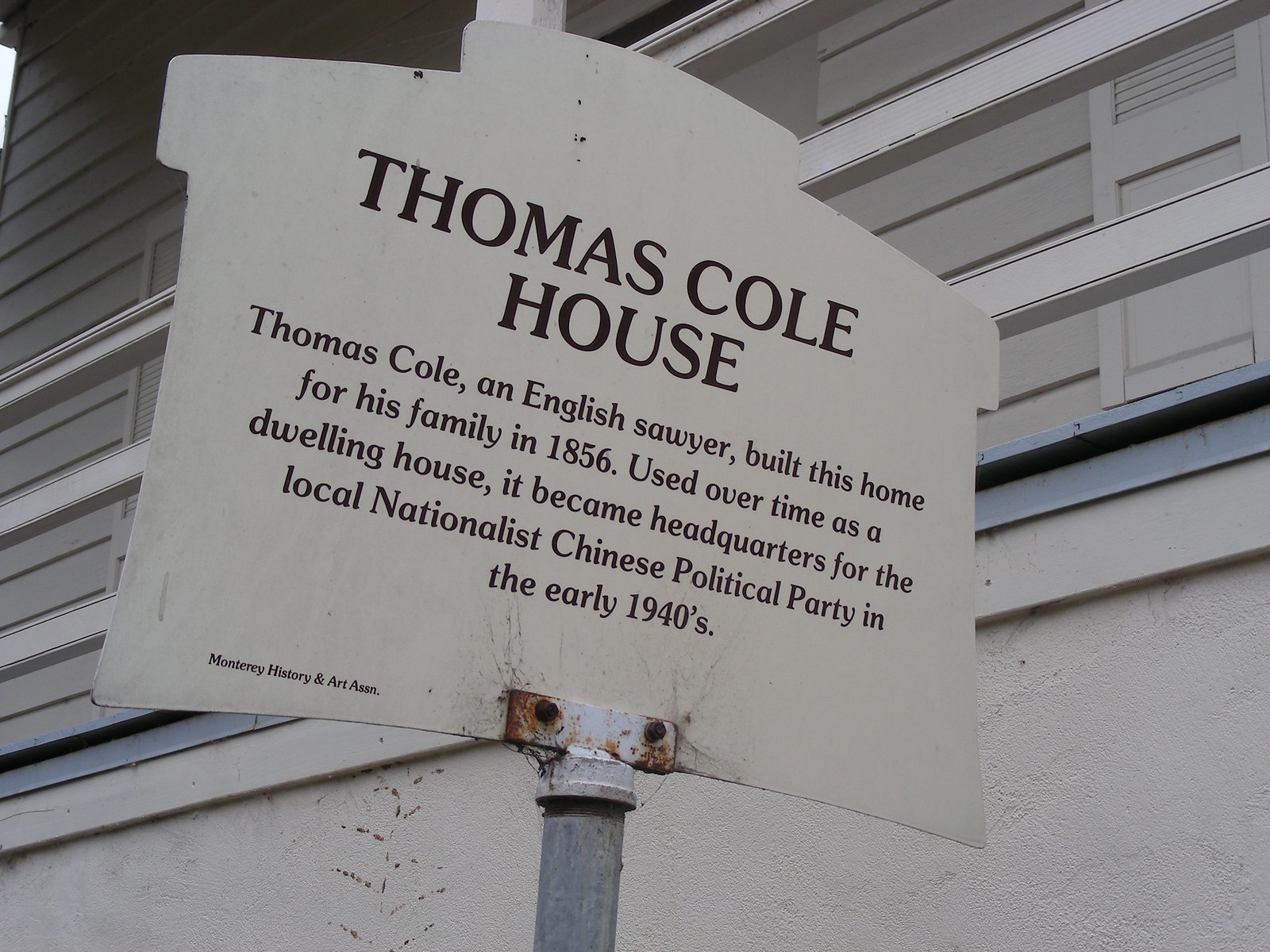This image depicts a thin metal sign mounted on the top of a silver pole. The sign is in the shape of a house and displays well-preserved black lettering against a white background. At the top, in large print, the sign reads: "Thomas Cole House." Below, in smaller print, it provides historical context: "Thomas Cole, an English sawyer, built this home for his family in 1856. Used over time as a dwelling house, it became headquarters for the local Nationalist Chinese political party in the early 1940s." The sign is held in place by bolts, noticeably rusted, and it bears a few scratches. On the bottom left corner, the sign credits the Monterey History and Art Association. The backdrop features a building with a white plaster wall at the bottom, transitioning to windows with closed blinds above. The windows have prominent white frames and may have white shutters, contributing to the overall historical atmosphere captured in the image.